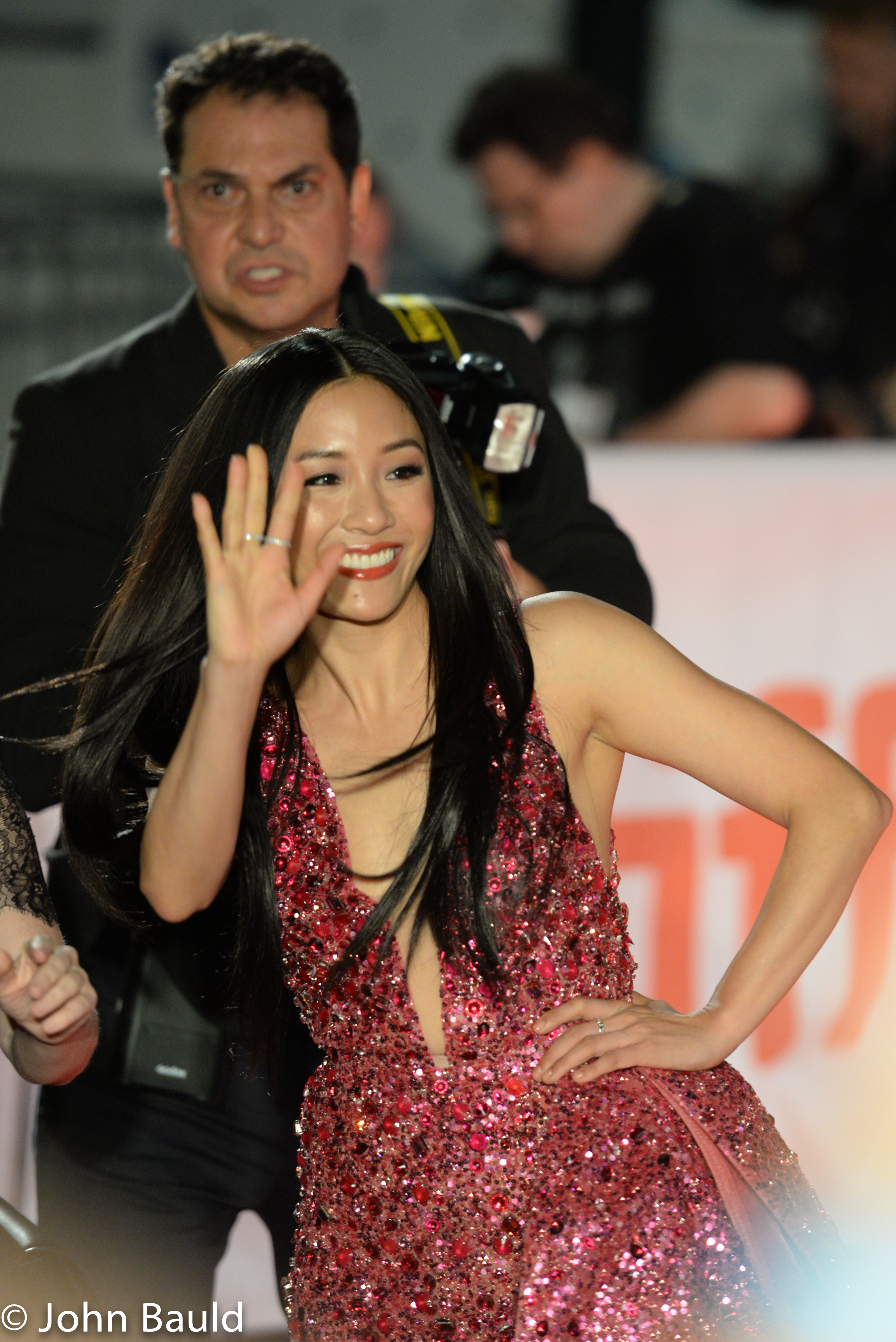In this vibrant photograph, a young woman dressed in a stunning, deep red, V-neck dress adorned with asymmetrical sequins and sparkling jewels extends her right hand in a wave, her fingers spread wide in a friendly gesture. Her left arm is bent at the elbow, with her hand resting confidently on her waist, drawing attention to the several elegant rings she wears. The woman, with her long, dark hair cascading around her face, smiles warmly, creating a sense of connection with the onlookers.

She stands in the center of the image, somewhat out of focus from what appears to be an official or public gathering setting, possibly a fan meetup. The background is blurred but reveals some context, including a wall at the bottom and figures, potentially camera crew, towards the top, bustling around. One distinct figure in the upper right corner is a man pointing towards the left side of the image, adding a dynamic element to the composition. Behind the woman, a stern-looking man in a black suit, possibly part of her security detail, has a strap, presumably for a camera, over his left shoulder. 

The color palette of the image is rich and varied, with shades of black, gray, white, yellow, pink, purple, silver, and orange, contributing to the vivid and lively atmosphere. Notably, the photograph is credited to John Bauld, with his copyright marked in white text at the bottom of the image.